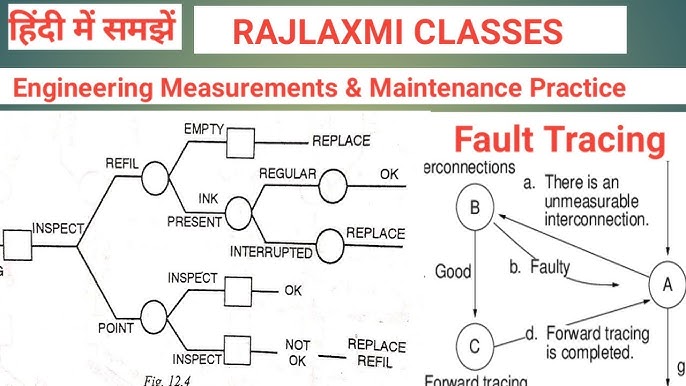This diagram, likely an educational flowchart used at a university or company in India, prominently features the label "Rajalakshmi Classes" and the title "Engineering Measurements and Maintenance Practice" in red text. At the top, there is a green rectangle followed by a white rectangle containing Indian characters on the upper left side. The flowchart starts with a square labeled "Inspect," which splits into two branches leading to "Refill" and "Point." These branches further divide into numerous interconnected pathways, labeled with tasks such as "Inspect," "Find," "Empty," "Present," "Ink," "Replace," and more. Embedded within the chart is a section titled "Fault Tracing" marked in red, showing a sequence with circles labeled A, B, and C, connected by arrows with additional descriptions indicating different states and interconnections, such as faulty conditions and completion of fault tracing. This detailed flowchart, marked as figure 12.4, visually maps out complex procedures and connections, illustrating various maintenance and measurement practices systematically.